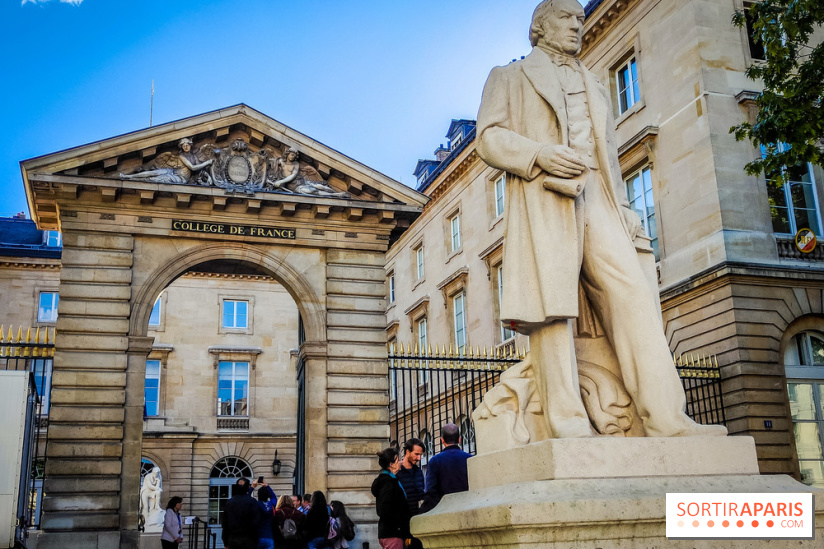This photograph captures the side corner of a stone and brick building identified as the Collège de France, illuminated under a clear blue sky. Prominently displayed above a stone archway leading to a courtyard is an inscription that reads "Collège de France." The architectural details reveal blue glass windows and a metal fence with spiked tops. Approaching the archway, we observe a large, human-like carved statue of a man in a long trench coat, holding papers and adorned with a bow tie around his neck, his curly hair cascading just above his shoulders. This statue features lifelike details, including a cloth at his feet and a subtle scowl on his face. Within the courtyard, another statue can be seen, depicting a seated figure deep in thought, with its head resting on its hand and elbow on its knee. Below the image, in the bottom right corner, is a watermark that reads Sortiraparis.com, firmly placing this evocative scene in Paris. The background bustle suggests visitors or perhaps a college orientation session, adding a lively human element to this historic and academic setting.